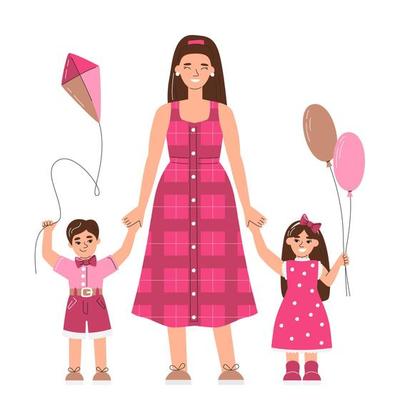This detailed cartoon image depicts a mother and her two children on a white background with no border or text. The mother, centrally positioned, wears a sleeveless plaid dress in shades of red and pink, adorned with white buttons down the front. She has long, straight brown hair with a small pink barrette. To her left, her young son is depicted with short brown hair and dressed in a pink shirt and dark pink shorts. His hands are raised; one is gripping the string of a diamond-shaped kite, which is divided into four sections colored dark pink, pink, light pink, and brown. His other hand clasps his mother's. On her right stands her daughter, wearing a polka dot jumper and pink boots, mirroring her mother’s long, straight brown hair and adorned with a pink bow. The girl beams with a wide smile, holding two balloons—one pink and one brown—in her right hand while her left hand holds her mother’s. Both the mother and her son wear brown shoes, highlighting a cohesive color palette of pinks and browns in their clothing and accessories.